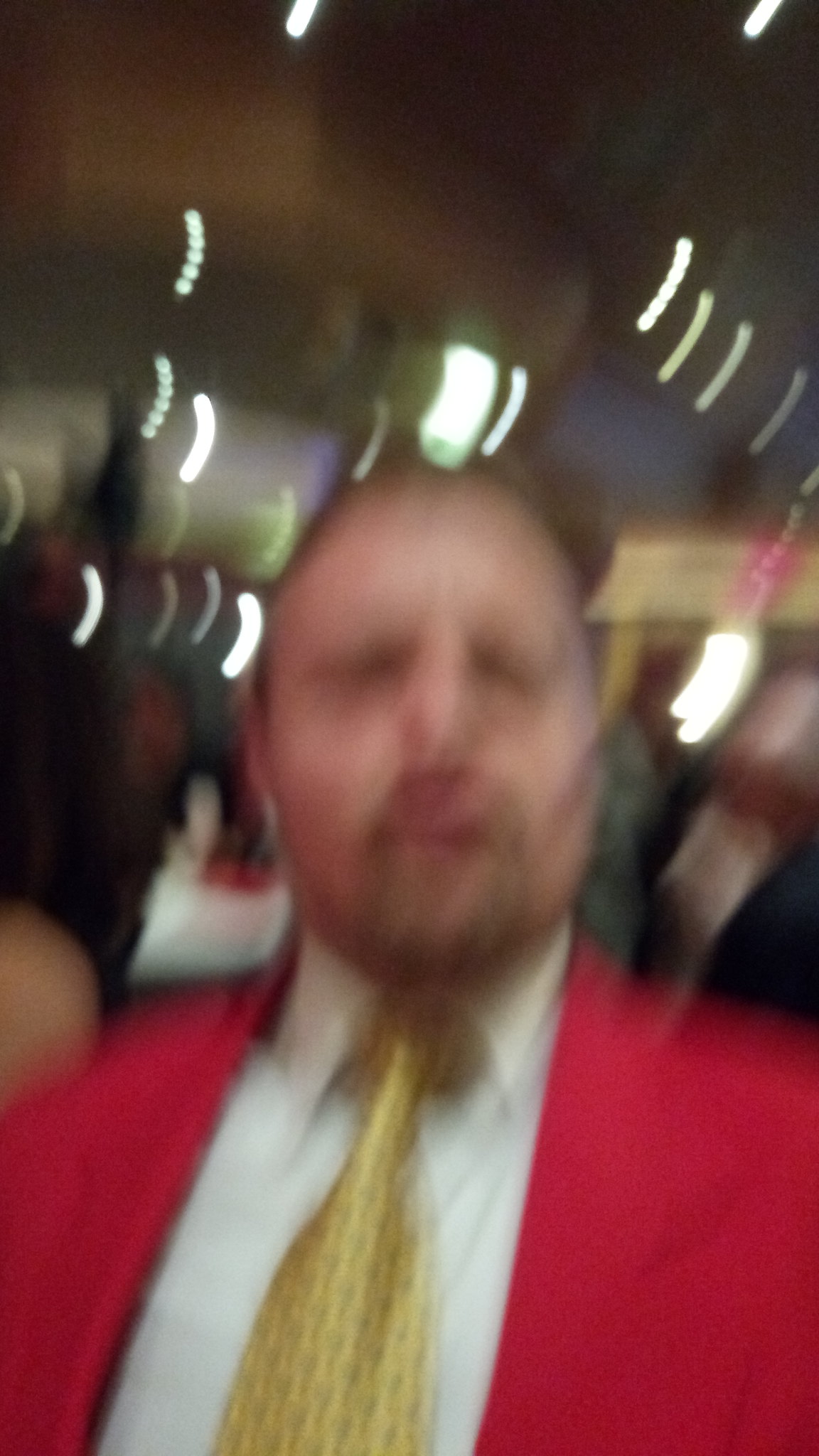A blurry selfie captures a man at a party, his expression reflecting a mix of confusion and curiosity. The man's light brown hair complements his mustache and beard. He's dressed in a striking red tuxedo with a golden patterned tie and a crisp white dress shirt underneath. Though the image is out of focus, you can make out the blurred background filled with decorative lights and indistinct figures. To the left of the man, the back of a brunette woman's head and shoulder are visible, while to the right, an older man in a tuxedo appears. Despite the lack of clarity, the man's attempt to take a selfie amidst the bustling party scene remains the focal point.